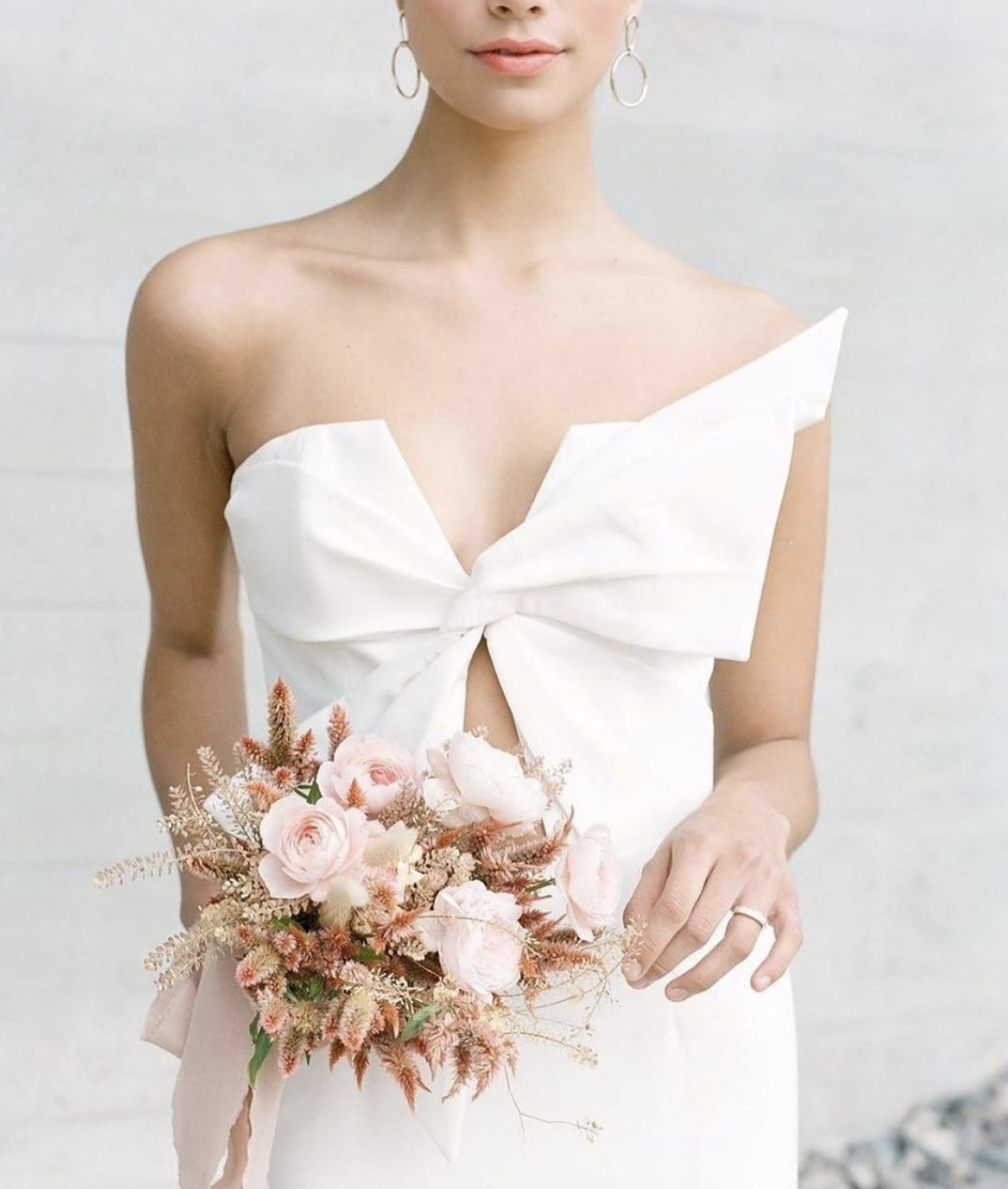This photograph captures a slender Caucasian woman, likely a bride, standing in front of a white brick-patterned wall. The vertical, rectangular image frames her from her nose down to about her thighs, omitting her eyes and the top of her head. She is adorned in a revealing shoulderless wedding gown that is white and features a large bow tied in the front. The dress covers her breasts with two little white cups and reveals a thin strip of her midriff before hugging her hips. Her shoulders are fully exposed. She accessorizes with silver hoop earrings, a wedding ring on her left hand, and light pink lipstick with her mouth slightly parted. In her right hand, she holds a beautiful bouquet of flowers, including white and light pink blooms, beige bushier flowers, baby's breath, feathery tan leaves, brown accents, and pink ribbons cascading down.